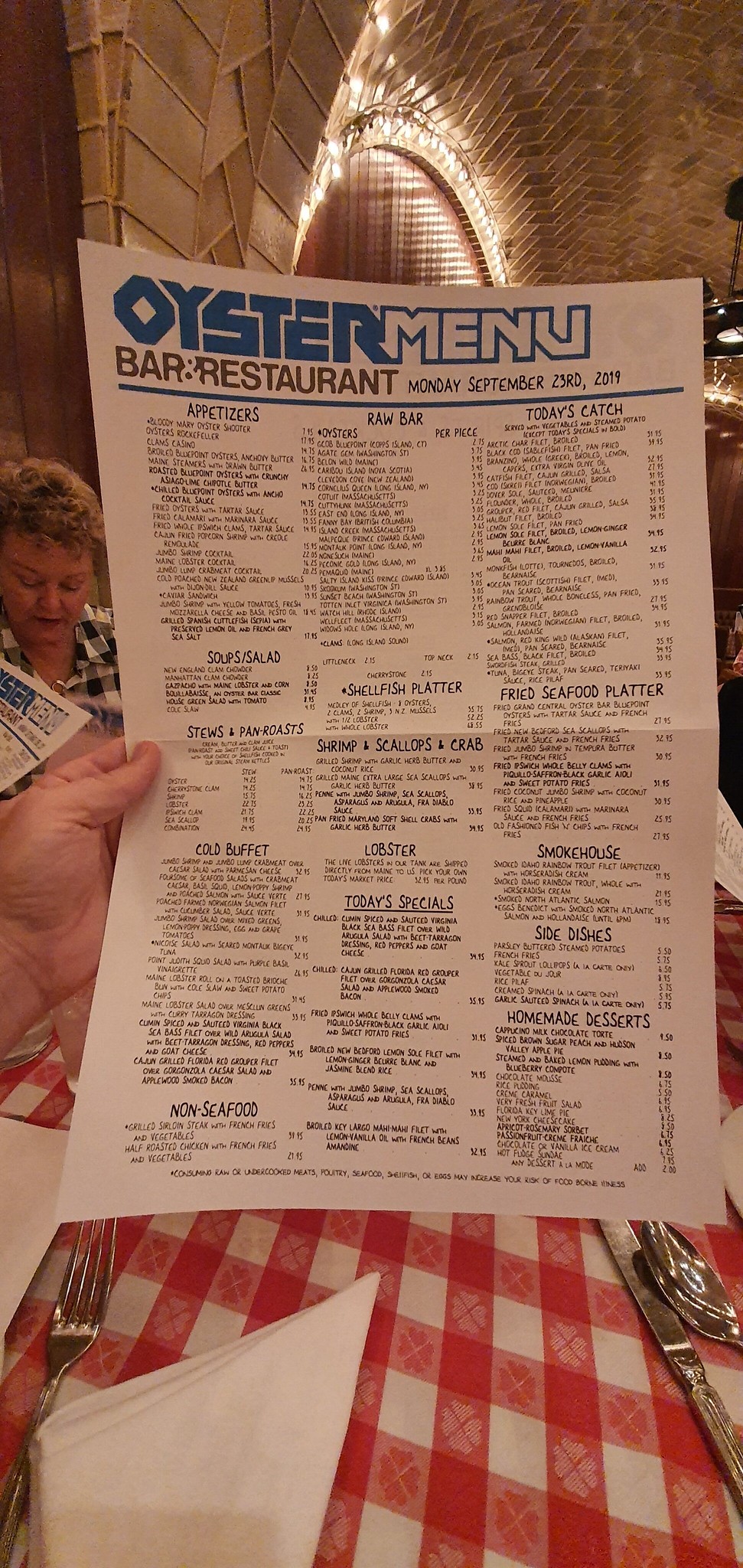This photograph captures a detailed view of a charming oyster bar and restaurant menu, held by a patron on Monday, September 23rd, 2019. The menu showcases a diverse selection of dishes, categorized into various sections including appetizers, a raw bar, today's catch, soups and salads, shellfish platters, fried seafood platters, shrimp and scallops, crab dishes, stews and roasts, non-seafood plates, today's specials, lobsters, smokehouse selections, side dishes, and homemade desserts.

In the background, a woman, identified as White, is engrossed in her own menu, while another diner, partly visible, does the same. This scene unfolds over a quaint table dressed in a red and white checkerboard tablecloth, adorned with small symbols resembling flowers or clovers. The table setting includes neatly arranged silverware and white napkins, creating a cozy and inviting dining atmosphere. Though several plates and dishes are scattered on the table, the text on them is too small to decipher. Overall, the image exudes a warm and rustic dining experience, capturing the essence of the restaurant's inviting ambiance.